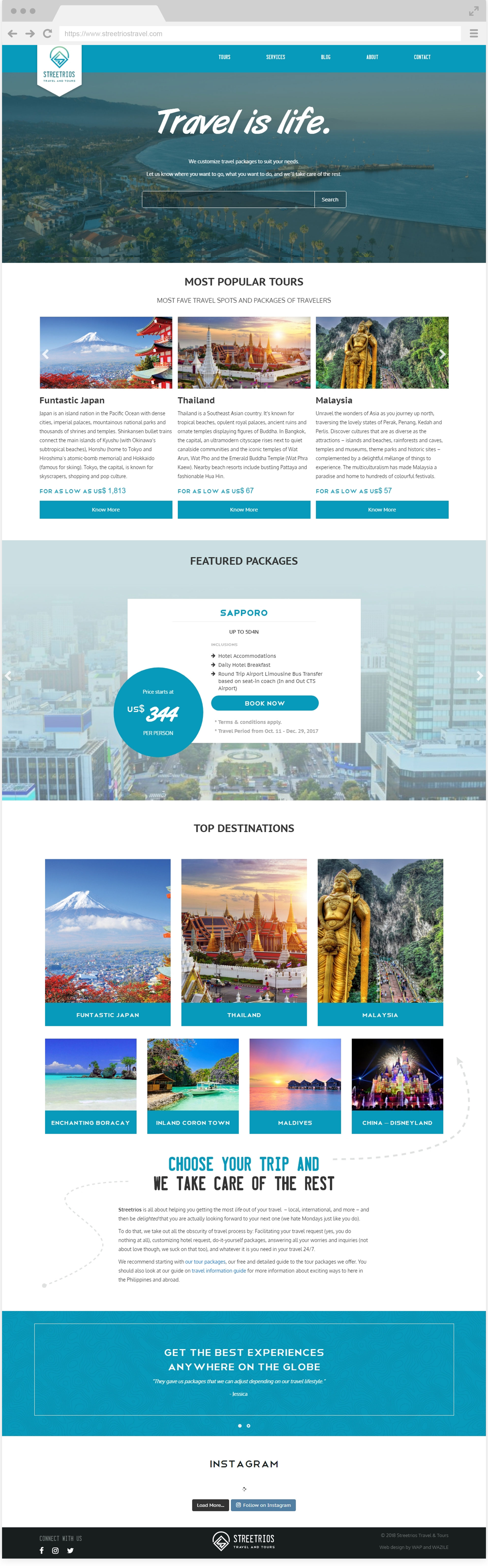This screenshot captures a travel agency's website, its background featuring a semi-transparent image of a picturesque port city with a large dock extending into the ocean. The main page is titled "Travel is Life" and prominently showcases popular tours with clickable country options. 

The first highlighted tour is "Funtastic Japan," featuring an iconic mountain and traditional Japanese architecture. Adjacent to this, a section labeled "Thailand" displays a beautiful sunrise or sunset scene, while the third column spotlights "Malaysia" with a gold statue.

Scrolling down, the page offers featured packages. One package is for Sapporo, Japan, priced at $344. This information is displayed in a rectangular shape with a small square in the middle labeled "Sapporo" and a blue circle to the left indicating the cost.

Further down, the page lists top destinations: Japan, Thailand, and Malaysia. It also mentions additional beach destinations such as China and the Maldives, among others that are difficult to discern. The tagline "Choose your trip, and we take care of the rest" encapsulates the site's promise to manage travel arrangements for their clients. The website is visually rich with images of the destinations, offering insightful glimpses into each tour.